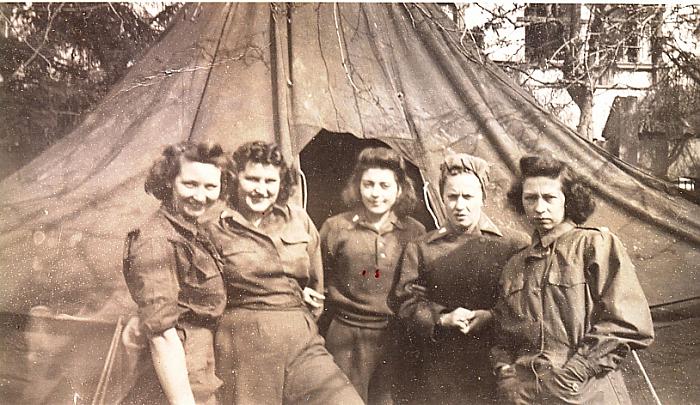This vintage black-and-white photograph, possibly from the 1940s during World War II, features five women standing in front of a large tent, with a building and some trees visible in the background. The women, who appear to be dressed in military uniforms, are all looking at the camera. Four of them are wearing military-style shirts and pants, while one has an army jacket adorned with military brass on the collar. Another woman is notable for her headgear, reminiscent of Rosie the Riveter, and has an unsmiling expression. The woman situated on the far right has a hairstyle similar to Queen Elizabeth's younger days and carries a serious frown. The rest of the women are smiling or have pleasant expressions on their faces. Their hairstyles are predominantly short bobs with curls in the front, a common style of that era. The photograph, with its sepia tone enhancing its vintage feel, captures a sunny day, casting bright light on the women's faces and the surroundings.